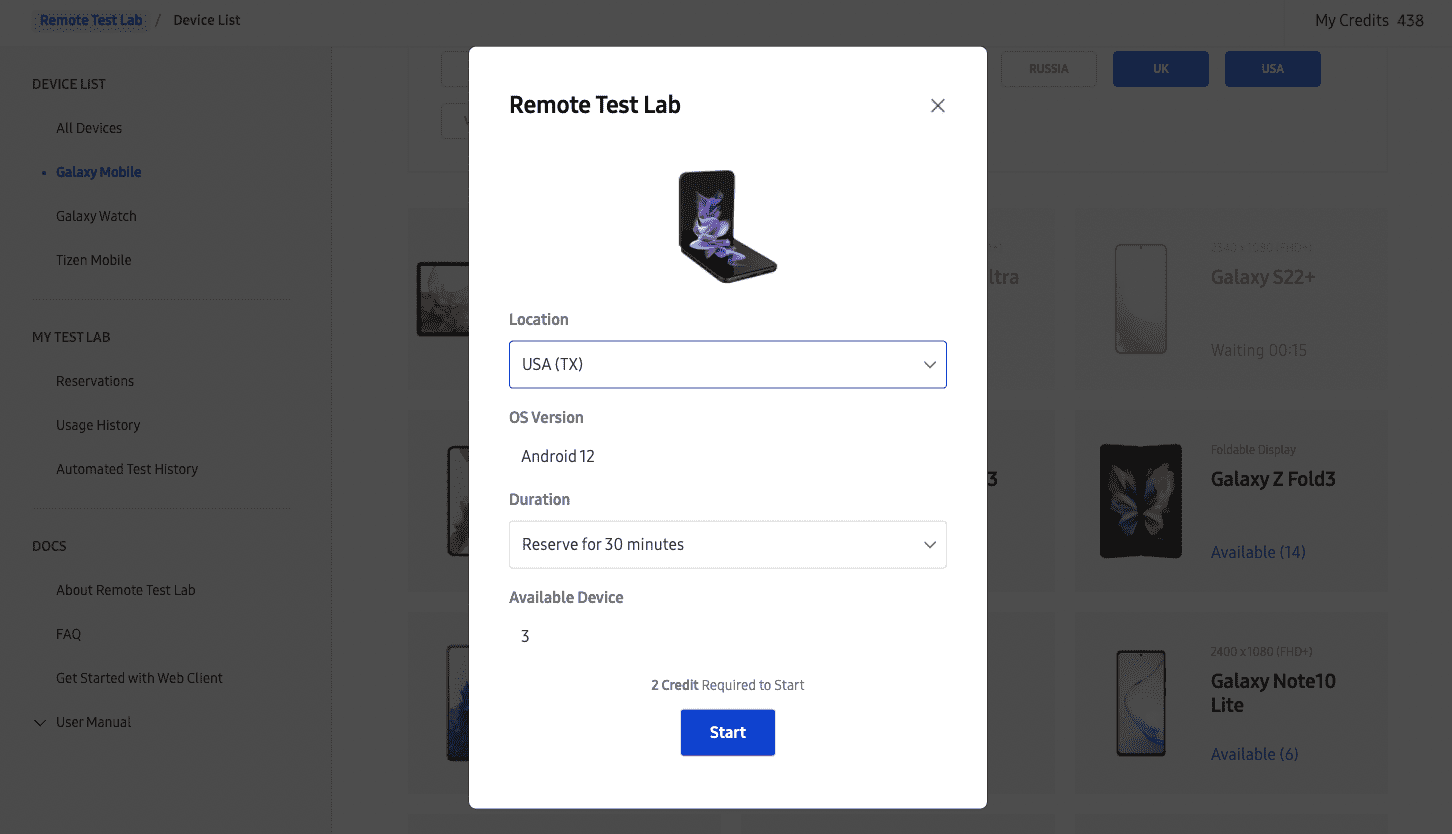The image depicts a web page with a medium to dark gray overlay, making the background text challenging to read. Despite the darkness, discernible text on the left sidebar includes: "Device list," "All devices," "Galaxy Mobile," "Galaxy Watch," "Tizen Mobile," "My Test Lab," "Reservations," "Usage History," "Automated Test History," "Docs," "About Remote Test Lab," "FAQ," "Get Started with Web Client," and "User Manual." 

Central to the image is a pop-up window on a white background titled "Remote Test Lab," with a close button ("X") in the top right corner. Below the title, there is an image of a folded cell phone. The section beneath this image includes a label "Location" with a dropdown box showing "USA (TX)." It is followed by "OS version," which indicates "Android 12." 

Next, there is a "Duration" section where a dropdown box reads "Reserve for 30 minutes." The text informed about the availability with "Available Device: 3" and the cost, "Two credits required to start." A blue button labeled "Start" is positioned at the bottom of the pop-up.

On the far right side of the background page, which is partially obscured by the dark overlay, there are images of various smartphones accompanied by their names: "Galaxy S22+," "Galaxy Z Fold 3," and "Galaxy Note 10 Lite," displayed sequentially from top to bottom.